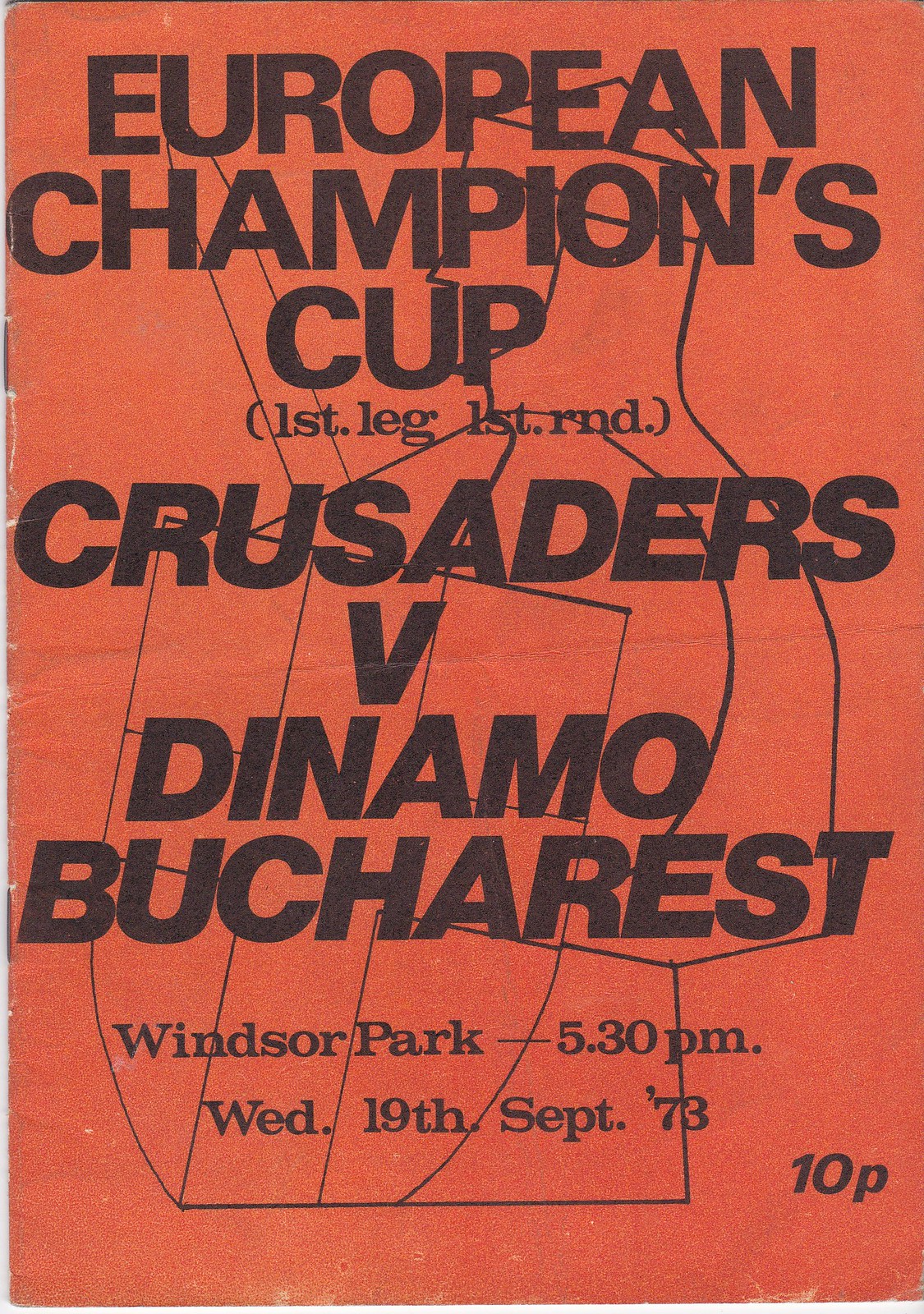This vintage red-hued poster, slightly faded with white speckles, features bold black text promoting a 1970s European Champions Cup match. The headline reads "EUROPEAN CHAMPIONS CUP" followed by "FIRST LEG, FIRST ROUND," and details the match-up: "Crusaders v. Dynamo Bucharest." Below, it specifies the venue and time: "Windsor Park, 5:30 p.m., Wednesday, September 19, 1973." In the bottom right corner, the entry fee is marked as "10P." The background includes abstract black line drawings, one resembling a shield in the bottom left corner, contributing to an artistic yet sporty aesthetic. Two staples on the left edge suggest this could be the cover of a booklet sports program.